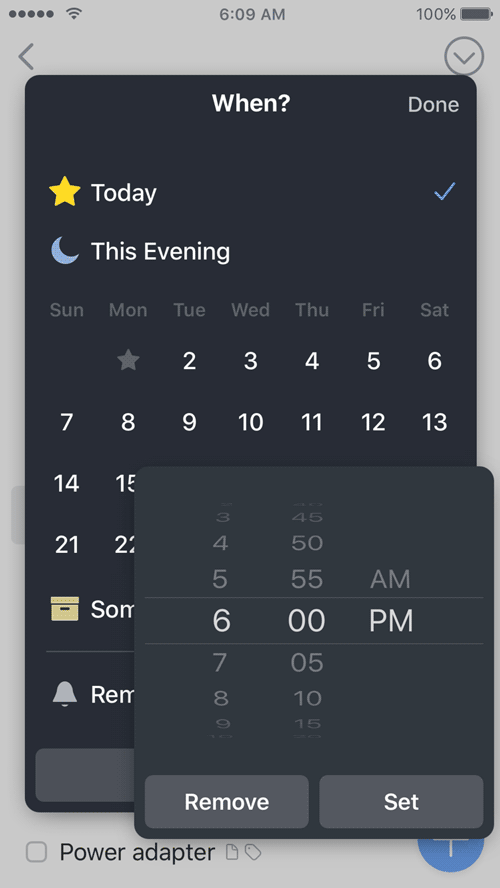Image Caption: 

The smartphone screen shows a detailed display of various notifications and prompts. In the top-left corner, there are five black dots next to a Wi-Fi symbol, displaying the time as 6:09 a.m. with a 100% battery life against a black background. 

The screen features several icons and messages arranged in a list format:
- A gold star symbol, labeled "Today," accompanied by a blue checkmark.
- A silver-blue moon icon labeled "This Evening."
- The days of the week listed horizontally: "Sunday, Monday, Tuesday, Wednesday, Thursday, Friday, Saturday," with a gray star underneath Monday.
- The numbers sequence: "2, 3, 4, 5, 6, 7, 8, 9, 10, 11, 12, 13, 14, 15, 21, 22."

Further down, there is a brown box labeled "Psalm" followed by the abbreviation "SOM." A notification icon showing "REM" appears next to it.

Several time stamps are displayed in a list format:
- 6:00 p.m. 
- Above that, 5:55 a.m.
- Above that, 4:50 
- Above that, 3:45 
- Below these times, additional timestamps are shown: 7:05, 8:10, and 9:15.

The screen also shows options to "Remove," "Set Power Adapter," and includes various miscellaneous icons, such as a folded-corner paper and a clothing tag. There is also a blue circle icon with a white 'T' in it.